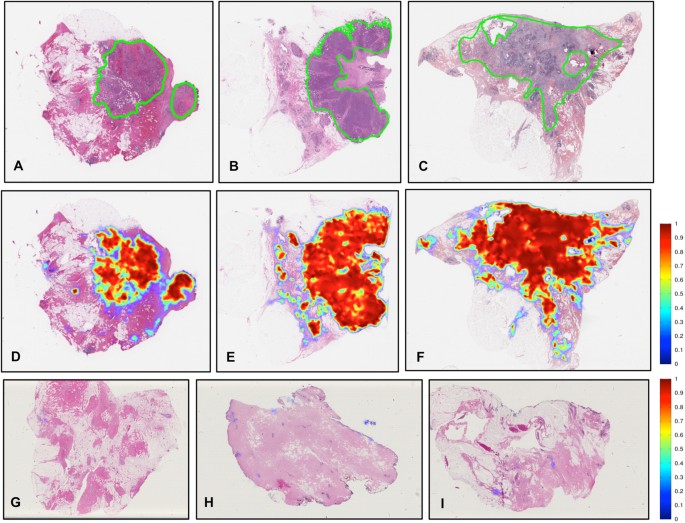The image is a compilation of nine distinct scan images, arranged in three rows and three columns, each bordered by a thin black line. The scans are labeled A through I, with labels positioned in the bottom left corner of each image. The visual content predominantly features a combination of colors—purple, pink, red, orange, and green—suggesting a type of scientific imagery, which might be radar, infrared, or hyper-spectral scans.

In the top row (A, B, C), each image showcases a reddish-purple mass, with some regions outlined in neon green. This green outline appears to encircle deeper purple areas within the masses. The middle row (D, E, F) exhibits similar purple masses, but with additional prominent red and orange areas inside the green-outlined sections, possibly indicating areas of increased heat or activity. The bottom row (G, H, I) presents softer, light-purple images which seem more transparent, and may depict magnified tissue sections or another form of detailed imagery.

The images on the top right contain a color key extending vertically, marked from blue to red. This key signifies a scale from zero (blue) to one (red), with increments of 0.1, likely representing data intensity or a specific measurement parameter. The overall setup, characterized by the intricacy of shapes and varied data presentations, hints at a scientific study, possibly medical or geological, aiming to highlight different attributes through color-coded visuals.